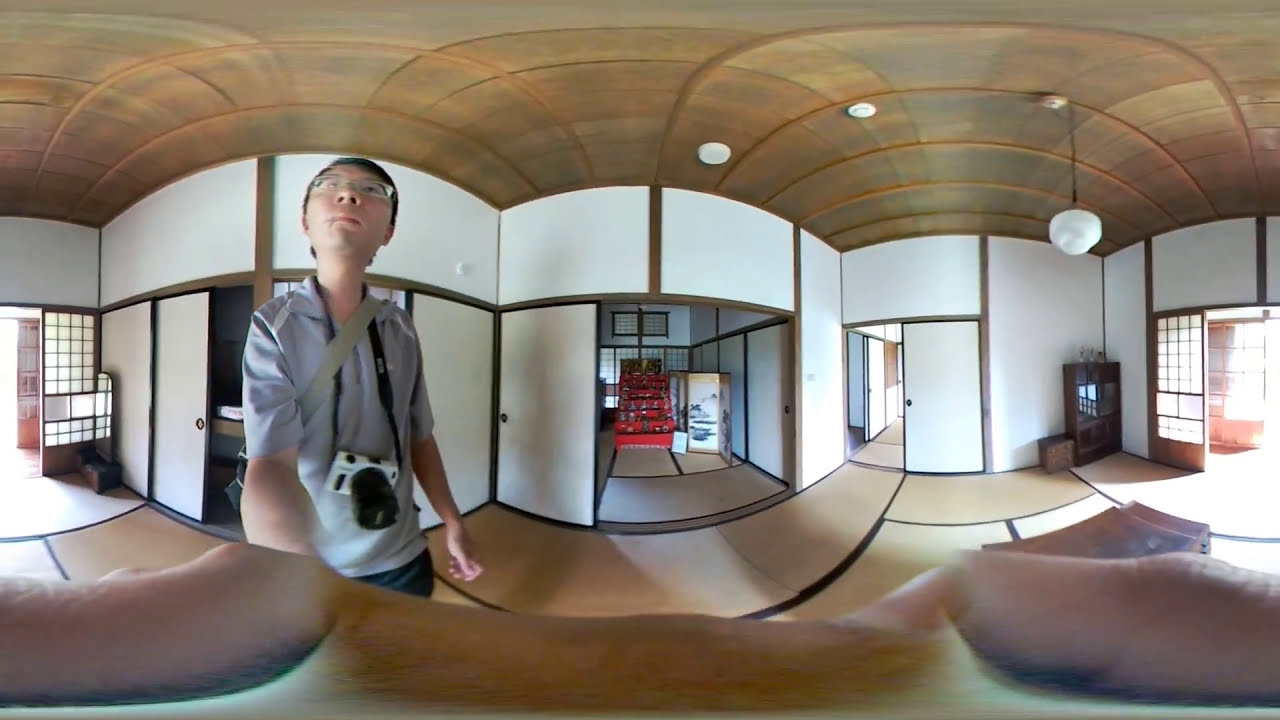The image depicts a slightly distorted, 360-degree view of an interior space, which appears to be influenced by Japanese architecture, characterized by several sliding paper doors. At the forefront stands a thin man, seemingly Asian with dark hair and silver glasses, wearing a grayish polo shirt and jeans. Around his neck hangs a camera with a black lens, a white body, and a black strap. The room in which he stands features brown floors with black borders and a brown ceiling adorned with two or three circular smoke detectors. To his right is a door, and in the center of the room, there’s a red display case or shelf that likely holds various products. Additional sliding doors lead to adjacent rooms, one on the right-hand side, giving an impression of partitioned sections within the building. Above, a single white light bulb hangs from the ceiling, adding a minimalist touch to the lighting. The overall setting is suggestive of a traditional Japanese house or perhaps a themed hotel or display area.